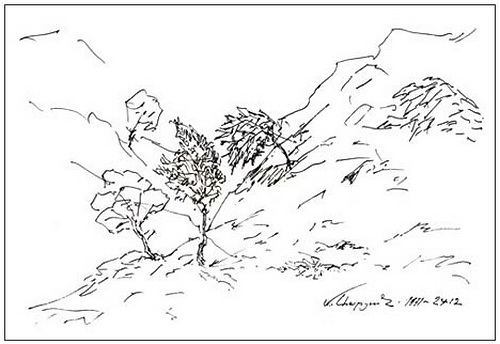The image is a simple yet detailed black and white line sketch of a mountainous landscape. The lines are uniform in thickness and predominantly straight, suggesting either pen or digital creation. The scene features two mountain peaks in the background, with the area between them left empty. In the middle of the image, slightly to the left, there are two types of trees: fuller, densely-leafed trees and fluffier, looser ones, making up a total of four trees. One of the fuller trees appears to be bending as if in the wind, while another is positioned higher up the slope. Additional sketching at the bottom right signifies rocky terrain and grass. A signature is present in the bottom right corner, accompanied by some numbers that are difficult to decipher, possibly a date or identifying marks. The entire composition is framed within a black rectangle, emphasizing the sketch's minimalist and illustrative nature.